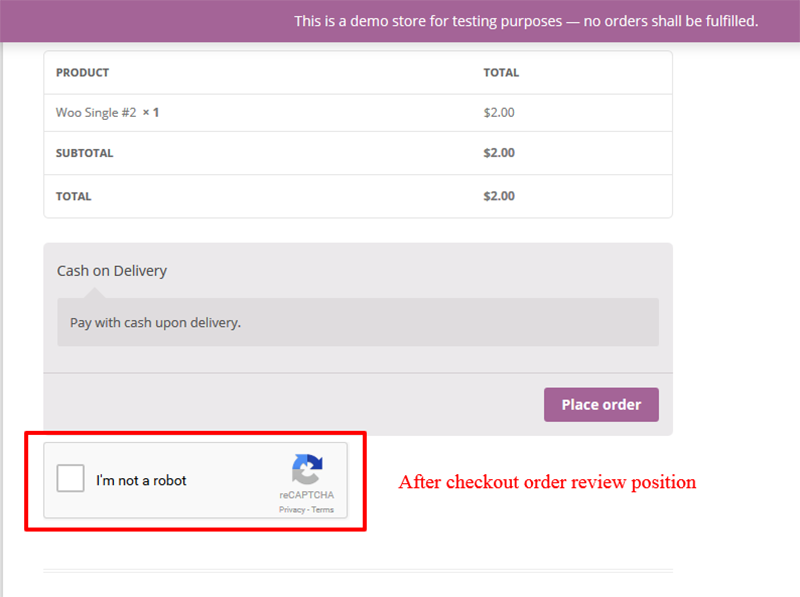The image is a screenshot from a computer, likely a desktop or laptop, displaying a web page with a primarily white background. Central to the image is a red box added post-screenshot, highlighting a specific section for emphasis. Beside the box, red text draws attention to the highlighted area. 

Within the red box, a "reCAPTCHA" checkbox is selected with the statement "I'm not a robot." Next to the checkbox is the reCAPTCHA logo, featuring three almost-connected arrows forming a near-circle in gray, blue, and dark blue.

Below the reCAPTCHA checkbox, text reads "after checkout order review position after checkout order review position." At the top of the page, a lavender banner states, "This is a demo store for testing purposes, no order shall be fulfilled," indicating that this is a mock checkout page for a fake product.